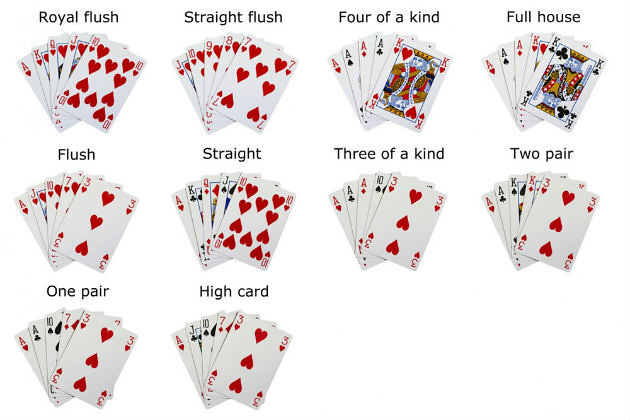The intended image failed to load, leaving a placeholder icon in its stead. This placeholder is a tiny green and blue square, commonly seen when an image download is unsuccessful. Despite this, I will proceed with describing the questions provided for evaluating the image's details. These questions prompt consideration of the image's first impression, object counts, text content, object positioning, subtle details, background, style, and color. The questions are listed on a yellow background, with each bullet point accompanied by different icons that relate to their respective inquiries. Time is running out as I document this information. Moving on to the next item.